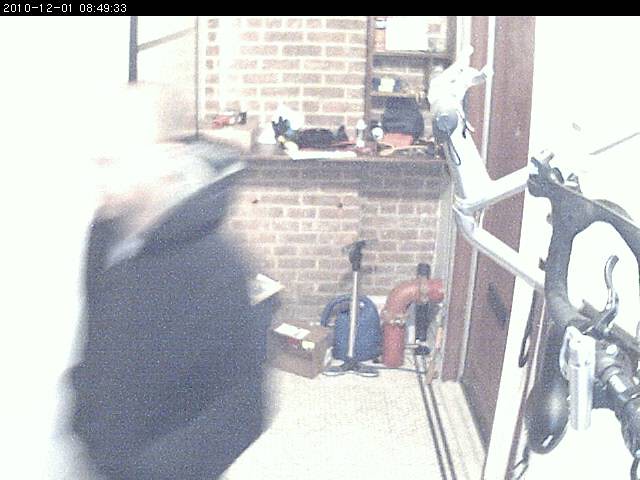This image, possibly taken indoors, exhibits a washed-out quality on the left side, leading to some blurriness. The background prominently features a red brick wall, adding texture to the scene. To the right, there is a brown door that suggests an entrance or exit.

Along the red brick wall, a shelf is visible, holding various items whose details are not discernible. Below the shelf, a large red pipe runs horizontally along the ground. Adjacent to the shelf, a blue object, potentially some boxes, adds a splash of color to the otherwise earthy-toned setting. 

In the right corner, there are additional elements: black components, possibly pipes, and white elements that also resemble piping, contributing to an industrial feel. A timestamp in the upper left corner reads "2010-12-01 08:49:33," providing context to the captured moment.

The lower left corner features a blurred, washed-out figure of a person. The individual appears to be a white male with closely cropped hair, dressed in a black coat, adding a human element to the otherwise static environment.